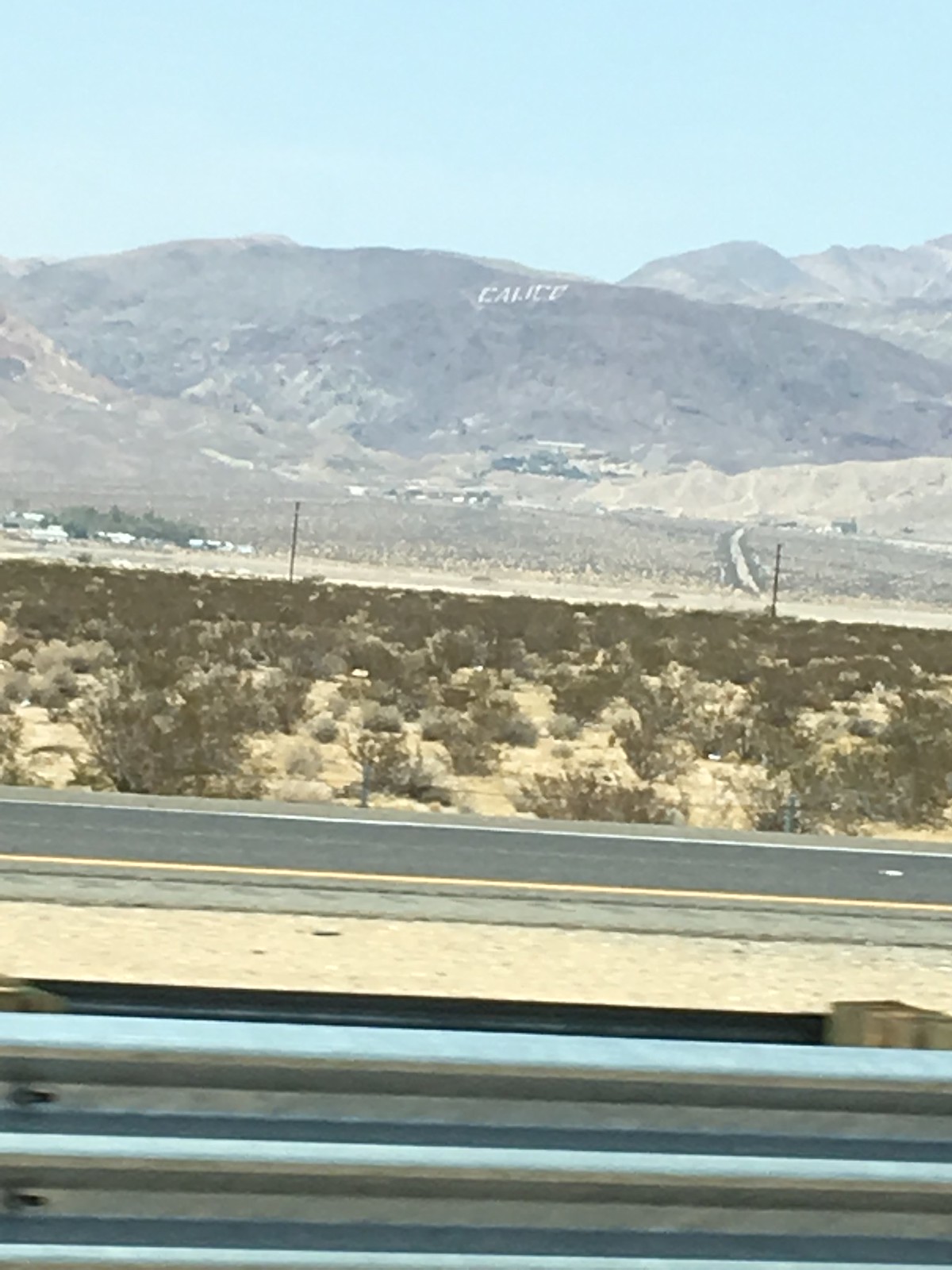The image appears to be a vintage-looking photograph of a desert landscape with a mountain range in the background. The colors in the photo are muted, giving it a slightly bleached-out appearance. In the far distance, the dark brown mountains have "Calico" spelled out in white on the mountainside, indicating a location name. Low, dark brown bushes dot the yellow desert sand, suggesting a dry environment with vegetation that requires minimal water. The foreground features a black paved road running horizontally with a steel guardrail that has a slight pale blue tint, likely to prevent collisions. Wooden electrical or telephone poles line the road, and the sky above is light blue, indicative of a daytime setting. Overall, the photograph captures the desolate beauty and stark elements of a desert, possibly in Arizona or New Mexico, with foothills and potential buildings visible in the distance.